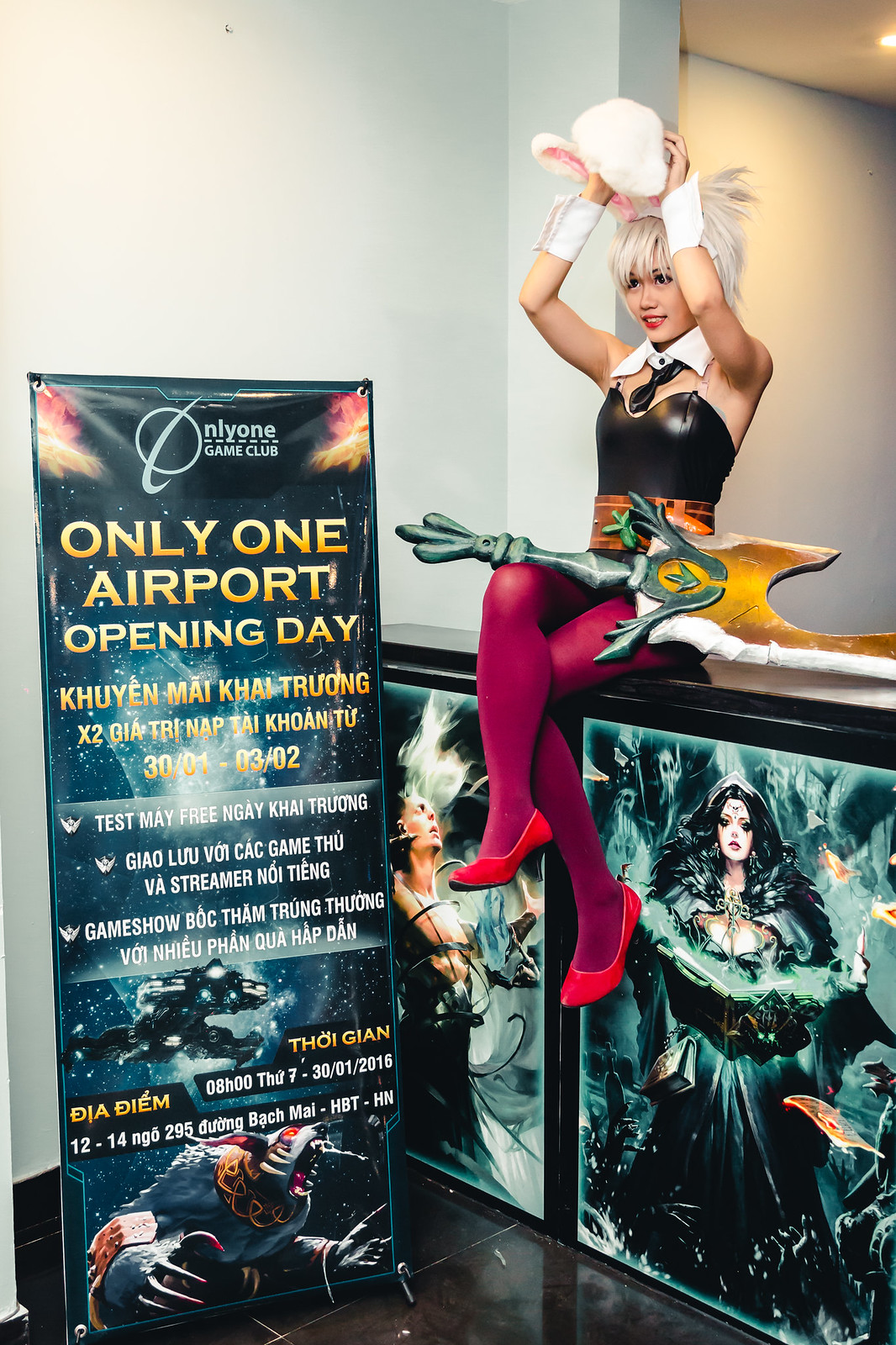In the photograph, a young woman adorned in a costume sits confidently atop a railing. She has a striking appearance with her short, silver-blonde wig and bunny ears, paired with a black halter top accentuated by an orange belt and complemented by purple nylons and red shoes. Across her lap rests a peculiar item resembling a sword or an unusual guitar. Behind her, a large, vibrant banner dominates the scene, proclaiming "Only One Game Club, Only One Airport Opening Day, Kuyanmai Kai Tuong, X2Gia Trinap, Tai Kwan Tu," followed by the date "30-01-03-032." The banner also bears more text in an unfamiliar Asian language, perhaps Vietnamese, Korean, or Thai. Among the detailed illustrations on the banner, a snarling wolf with human-like hands stands out at the bottom, and above it, a spaceship is depicted against a night sky. The image exudes a sense of a gaming or cartoon-themed event, possibly related to cosplay, suggested by the fantastical attire of both the woman in the photo and the characters on the banner.